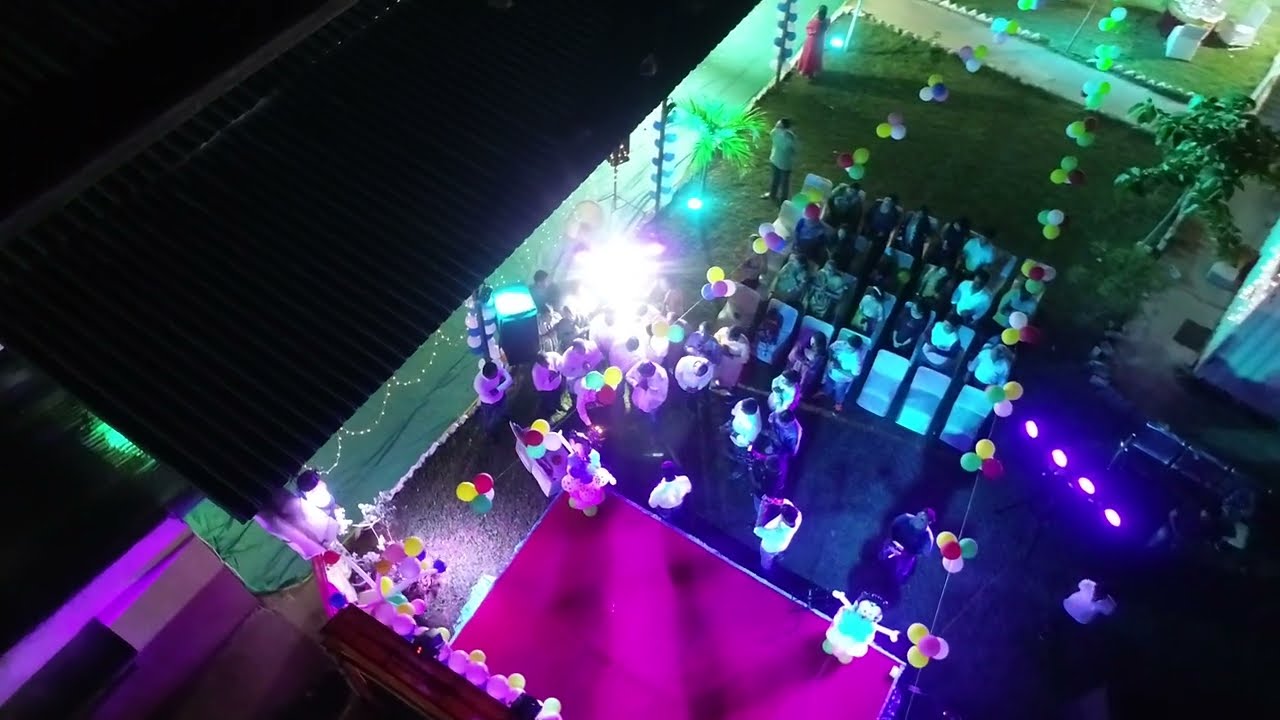The image depicts an aerial view of an outdoor nighttime celebration in a courtyard adjacent to a building with a metal roof awning visible on the left side. The scene centers around a brightly lit stage, which appears to be red in color, situated at the bottom of the image. The stage is flanked by clusters of balloons strung along clotheslines, hanging both around the edge of the stage and above the audience. The area is further illuminated by a series of purple lights to the right and blue lights to the left. Towards the top left corner of the image, part of the building’s black roof is visible.

In front of the stage, there are approximately four rows of white chairs, each row containing around seven seats, with about 20 people seated and focused on the performers on stage. The performers, numbering approximately six or seven, seem to be engaged in either singing or playing musical instruments. A particularly bright light is prominent in the middle of the image, casting a strong illumination over the scene. The presence of additional white lights hanging under the metal roofing enhances the festive atmosphere. The combination of balloons, colored lights, and the arrangement of the audience conveys a lively party or celebration taking place in the courtyard.